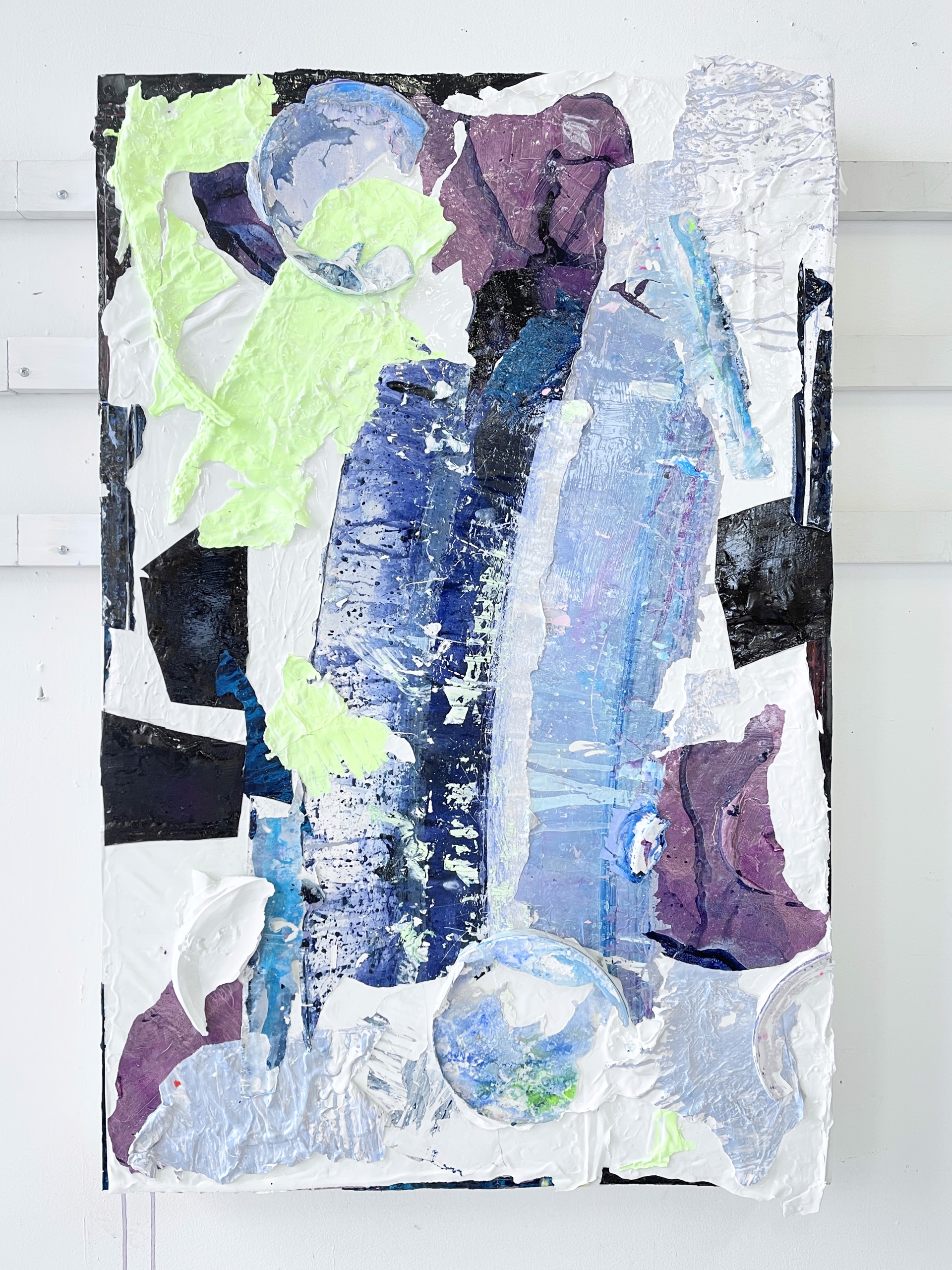The image portrays an abstract painting mounted on a white wall that features three thin horizontal wooden slats. The painting, which uses a mix of pastel and acrylic paints, showcases a white background with various smudged and textured brushstrokes. The color palette includes dark and light shades of blue, black, purple, lilac, gray, mint green, and scattered yellows. The canvas reveals intricate details with raised brushstrokes and gapped areas, giving it a textured appearance. Despite the chaotic, geometric arrangement of the colors, notable circular shapes can be observed in the lower part and upper left corner of the artwork, reminiscent of Kandinsky's style but without any discernible shapes. The focal point of the image is this detailed, framed piece of abstract art.